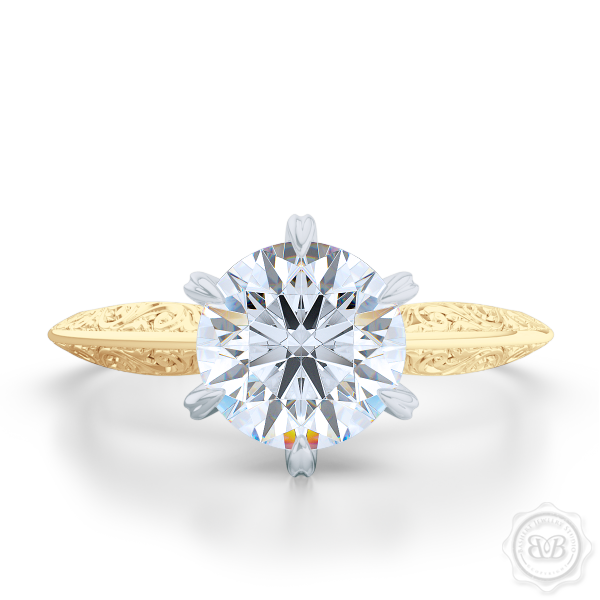The close-up image showcases a luxurious diamond ring, likely an engagement or wedding ring, placed on a blank white background. The ring features a prominent, circular diamond held in place by six silver-colored prongs. The band, made of gold, displays elaborate, naturalistic, and intricately etched designs. A distinctive thick gold band runs down the center of the band. The ring's aesthetic is enhanced by faint colors of blue and brown within the intricate carvings. At the bottom right of the image, there is a subtle watermark resembling two cursive B’s, back-to-back, surrounded by faint, illegible writing along the inner rim, indicating the jeweler's mark.